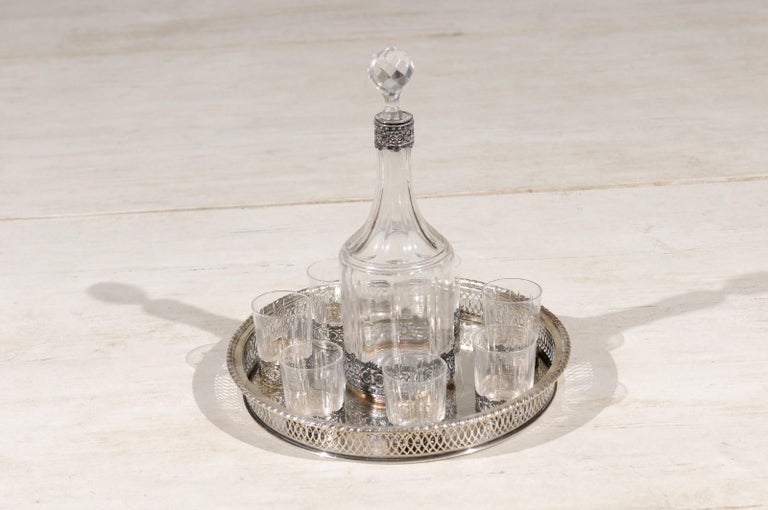The image depicts a miniature set, featuring a circular, silver serving tray with detailed, filigree edges that displays signs of wear and rust. The tray is placed on a light-colored floor, which appears to be either white marble or beachy white wood-look tile. Central on the tray stands a glass decanter with a distinctive, diamond-patterned crystal stopper and a black rim around its neck. The decanter casts shadows on both the left and right sides, suggesting lighting from two directions. Surrounding the decanter are six clear drinking glasses. Both the decanter and glasses have matching black lace borders at their bases, completing the elegant yet slightly aged aesthetic of the arrangement.